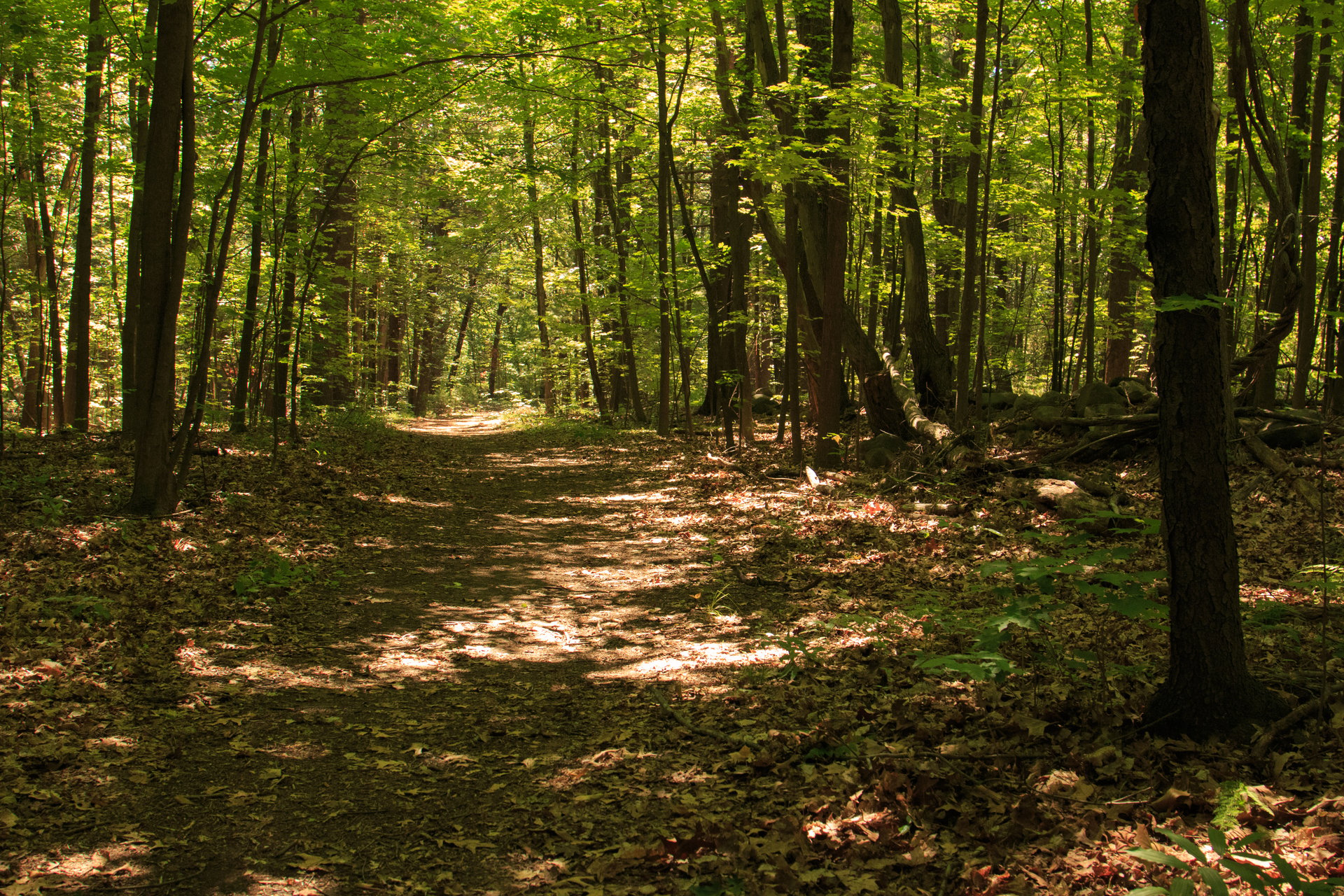This is a color photograph of a forest in landscape orientation, capturing a serene scene of a path meandering through dense woods. The viewer stands at the widest part of the trail, which narrows and recedes into the distance, creating a feeling of depth and invitation. Dappled sunlight filters through the canopy above, casting splotches of light and shadow patterns on the ground. The ground itself is a blend of brown tones, covered with fallen leaves and debris, signifying a natural, untrodden path rather than a well-defined road. Surrounding the path, numerous thin tree trunks stretch upwards alongside a few larger ones, including a dominant trunk on the bottom right that extends out of frame. The trees and foliage are rich with varying shades of green and brown, creating a harmonious and immersive woodland scene. No text or people are present, focusing solely on the natural beauty and tranquility of the forest. The image exudes a quiet realism, capturing the essence of being deep in the woods, shielded from the sky by the dense tree cover.